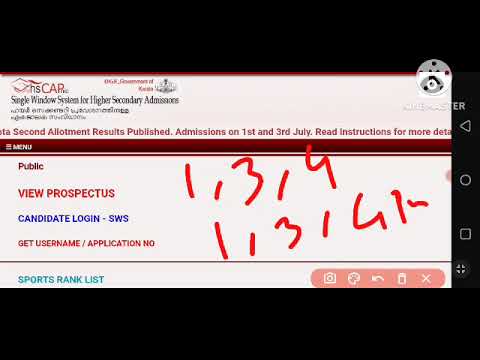This image is a detailed screenshot of an online application system, specifically titled "Single Window System for Higher Secondary Admissions" at the top left corner. It features a white rectangular section with a red line across the top, set against a black vertical background. Key details within the white section include: "Second Allotment Results Published" and "Admissions on 1st and 3rd July," followed by the instruction "Read instructions for more details."

Below this are several clickable options in different colored fonts: "Public View Prospectus," "Candidate Login," and "Get Username/Application Number" in blue, and "Sports Rank List" in teal. Overlaid on the image, there's handwritten text repeating the sequence "1, 3, 4, 1, 3, 4, 1." Additionally, there is an Instagram camera icon present.

On the right-hand side of the image, the phone’s navigation buttons (back, menu, and app buttons) are visible, indicating that the phone is held horizontally. The overall setting of the image implies a notice or results page for higher secondary school admissions, with key admission dates and procedural instructions prominently displayed.